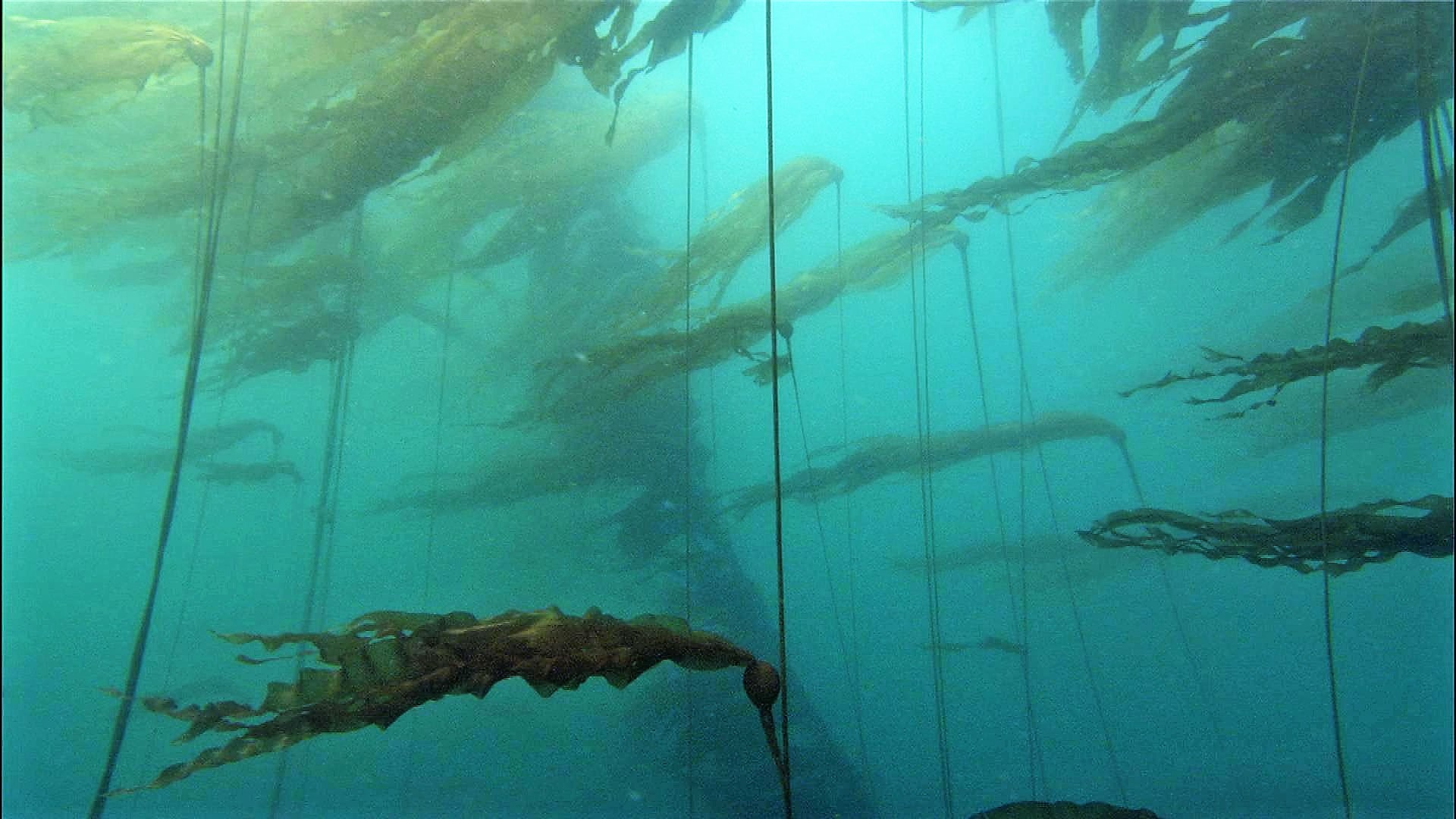The photograph captures a serene underwater scene in a blue medium-colored, slightly murky ocean. Light filters through the translucent water, illuminating a cluster of seaweed-like plants that are predominantly green. Attached to a large green bulb, these plants feature long, wavy, tentacle-like strands that flow to the left with the ocean current. Most of these strands are thin and solid, but one in the background is distinctive, covered with tendrils from top to bottom. The rectangular image, whose length is twice its width, showcases these plants arranged horizontally, with prominent sections in the top left and right corners as well as spread along the bottom. The plants, resembling grassy weeds, create a captivating underwater tableau, accentuated by the interplay of light and shadow in the ocean depths.